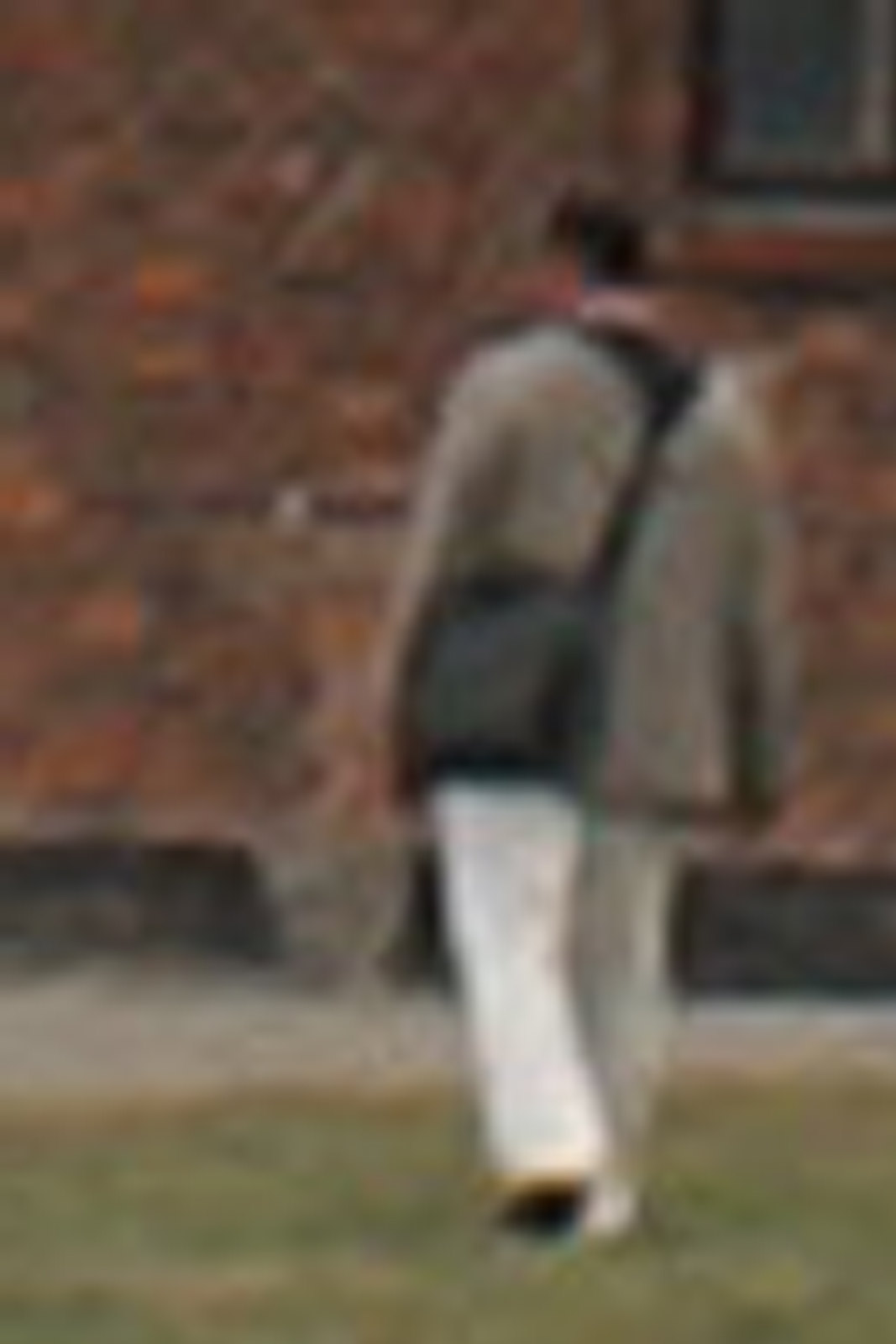The image depicts a heavily pixelated and blurry scene, appearing to have been significantly enlarged beyond its original resolution, thus compromising its quality. In the center, a person is seen walking away from the camera, with only their back visible, making it difficult to determine their gender. The individual is clad in a light gray top and loose white pants and is carrying a satchel resting against their side, with their arm casually placed on it. 

Ahead of the person, there stands a brick building with dominating hues of red and light red, culminating in a black base. The person appears to be walking on a grassy expanse, and they sport black shoes, though only their left shoe is clearly visible due to the motion of their stride—one foot on the ground and the other slightly raised. In the top right corner of the image, there is the faint outline of what seems to be a rectangular window frame, though the extreme pixelation makes it ambiguous.